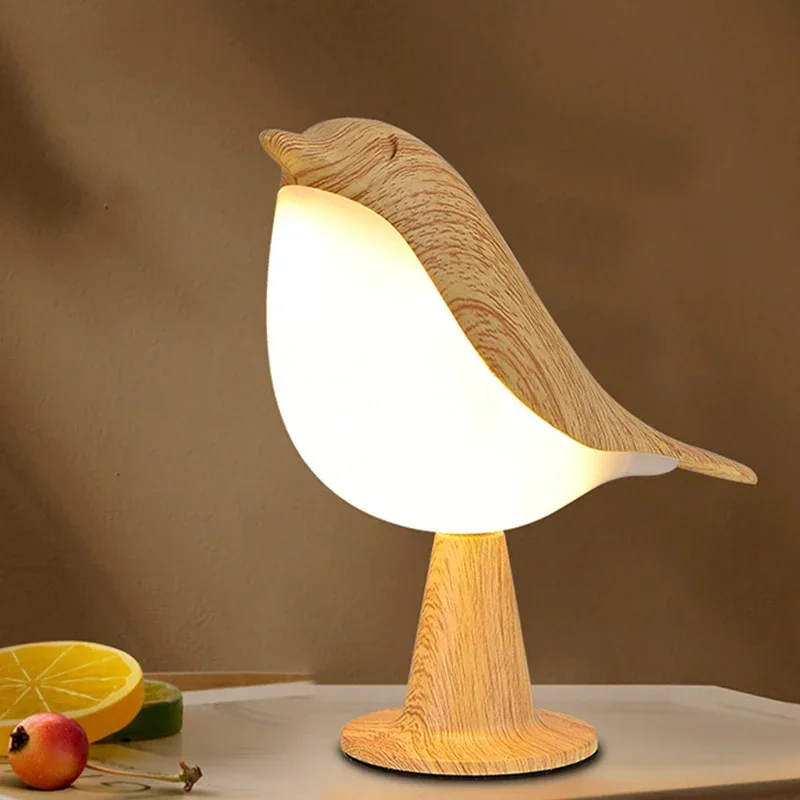The image features a detailed wooden carving of a bird, likely a dove, perched on a round, tapered wooden pedestal. The top part of the bird showcases the natural tan-colored grain of the wood, including a small slit for the eye and a modest bill. The bottom portion of the bird is white with a hint of yellow and a touch of purple, glowing brightly as if illuminated from within, suggesting it could function as a lamp. The intricate pedestal supports the bird and the entire piece rests on a grayish metallic surface. The background consists of a neutral brown wall. In the foreground, to the front right of the bird, there is a realistic-looking arrangement of fruit, including a slice of lemon, lime, and a cherry with a yellow tinge, hinting at an artificial quality to their appearance.